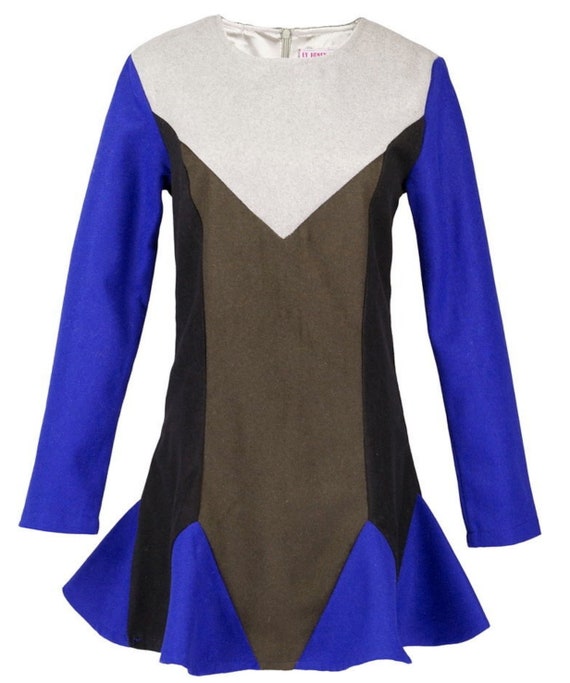The image depicts a short, long-sleeved uniform, potentially for activities like cheerleading, ice skating, or dancing, suspended against a white background as if it's being showcased for a website. The garment, which appears to be form-fitting and designed to sit high on the thighs, combines several colors and patterns. The torso features a light beige or very light gray section that forms a triangular point from the shoulders downward. This section contrasts with the shiny black material that covers the middle part of the dress. The skirt part flares out slightly and incorporates multiple blue triangular pleats or extensions, matching the long navy blue sleeves. At the back, a zipper is visible above the collar line, indicating it is used to fasten the dress. Inside the garment, a small white tag with red text can be seen, though the writing on the tag is too small to be deciphered.